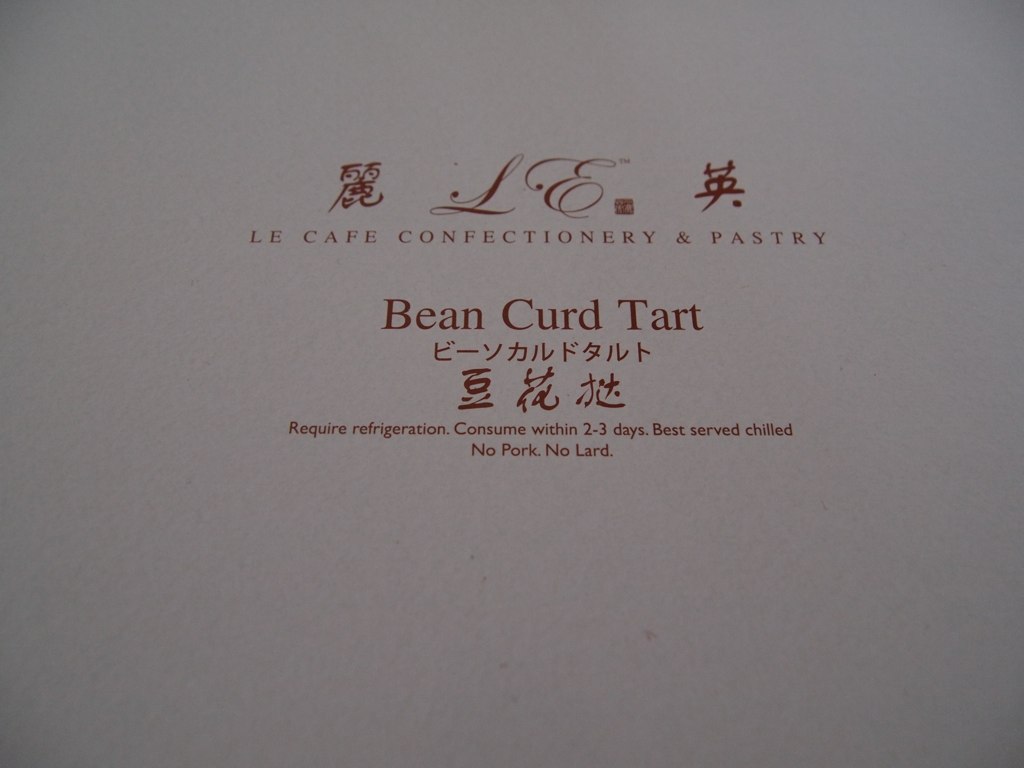This close-up photograph captures the side of a white packaging box, fading to a solid white, nearly gray background. Dominating the top center is a cursive, red "LE" logo flanked by Asian symbols. Beneath the logo, in bold capital letters, it reads: "Le Cafe Confectionery and Pastry." Centered below this, the product name "Bean Curd Tart" is displayed in a prominent serif font, followed by translations in Japanese and Chinese. At the bottom of the text block, smaller red print advises: "Require refrigeration. Consume within two to three days. Best served chilled. No pork. No lard." The minimalist design and straightforward layout suggest this text is typical for bakery packaging.